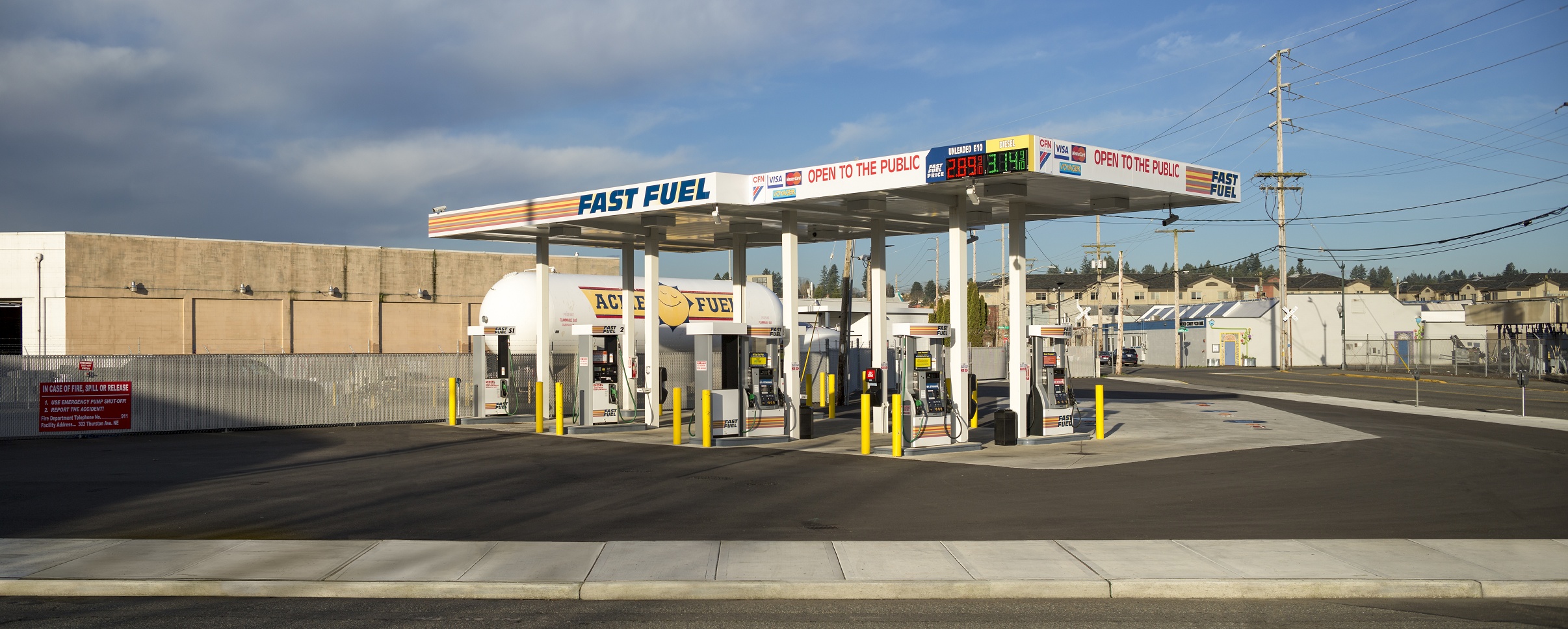The image depicts a well-maintained gas station situated in an urban or industrial environment. The station features a pristinely paved dark asphalt surface with smooth, gray concrete walkways encircling it. It has four to five standard gas pumps, each protected by tall yellow cylindrical concrete barriers.

Above the pumps, a large overhang displays the text "FAST FUEL" in blue on a white background, followed by "OPEN TO THE PUBLIC" in red. The pricing information indicates unleaded gasoline at $2.89 in red and diesel at $3.14 in green. Supporting the overhang are rectangular columns.

In the background, there is a large cylindrical fuel tank labeled "ACME Fuel" in blue text on a yellow background. A tan-colored warehouse and other industrial buildings, possibly warehouses or factories, are visible further back, along with some apartment buildings and numerous trees. The sky is bright blue with puffy white clouds, adding to the clean and freshly built appearance of the gas station. Additional details include a red sign on a fence, white buildings in the distance, and some telephone wires running across the scene.